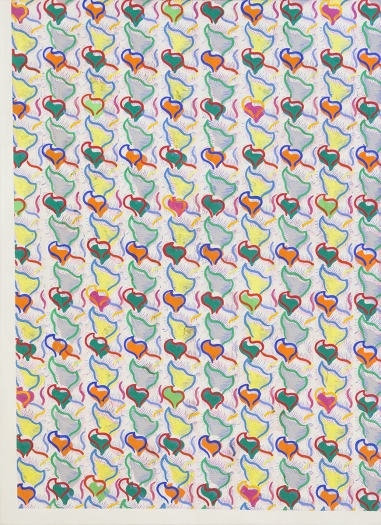This image features an abstract artwork, possibly created with ink, colored pencils, or paint. It is a vertically-oriented rectangle with no text, comprised of a pattern of curvy, triangle-like shapes that resemble hearts. The composition includes 10 vertical columns and 10 horizontal rows. Each column contains shapes that are alternately large and small, almost resembling tornadoes or seashells, giving the appearance of distorted hearts.

The distinctiveness of the artwork lies in its varied yet harmonious use of color. The colors featured include shades of green, pink, light blue, yellow, orange, and magenta. The coloration of each column varies, creating a visual rhythm across the piece. For instance, one column might alternate between reddish-pink and yellow, while another might switch between light green, lime green, and grayish-green. Additionally, swirls in red and green are scattered throughout the design, contributing to the intricate detail and overall unity of the piece.

Each repeated shape is imbued with slight variations in color, providing a sense of individuality while maintaining a cohesive pattern. The alternating colors and differing heart shapes create a mesmerizing effect, drawing the viewer's eye vertically down through the complex yet orderly design.